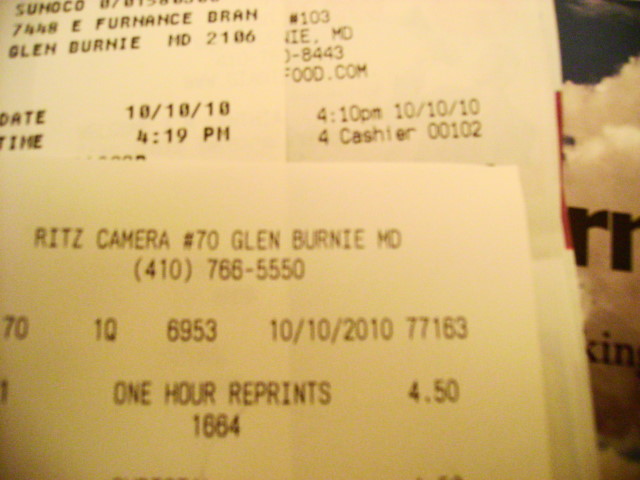The photo features three partially visible receipts under a yellowish lighting. Dominating the foreground is a receipt from Ritz Camera No. 70 in Glen Burnie, Maryland, dated October 10, 2010, detailing a purchase of one-hour reprints for $4.50. Positioned in the background on the left is a receipt from Sunoco, also dated October 10, 2010. Slightly obscured and to the right, another receipt appears, but the store's name is indiscernible, though it shares the same date.